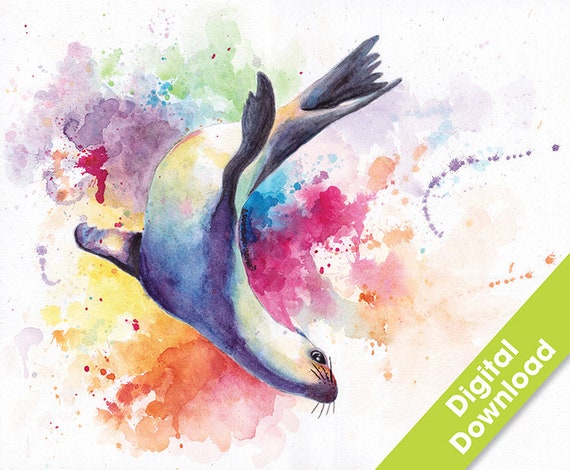This is a detailed watercolor painting of a seal, showcasing a mix of vivid hues and delicate brushwork. The central figure is a white seal with gray and black accents, distinguishable by its whiskers and black eyes. The seal appears to be executing a backflip, creating a dynamic 'C' shape with its body, head pointed downward and tail arching upwards. Interestingly, the underbelly, although primarily white, is tinged with shades of blue, pink, and yellow from the colorful background that bled onto it. The backdrop bursts with an array of colors, including dark pink, purple, green, blue, orange, yellow, and red, spread in a cloudy, almost dribbled aesthetic, giving the impression that paint was spontaneously thrown onto the white canvas. Adding a finishing touch, in the bottom right corner, a light green ribbon with white lettering states "digital download." There are no other texts in the piece, which merges a playful splatter of colors and a lifelike pose to create a visually engaging and lively image.